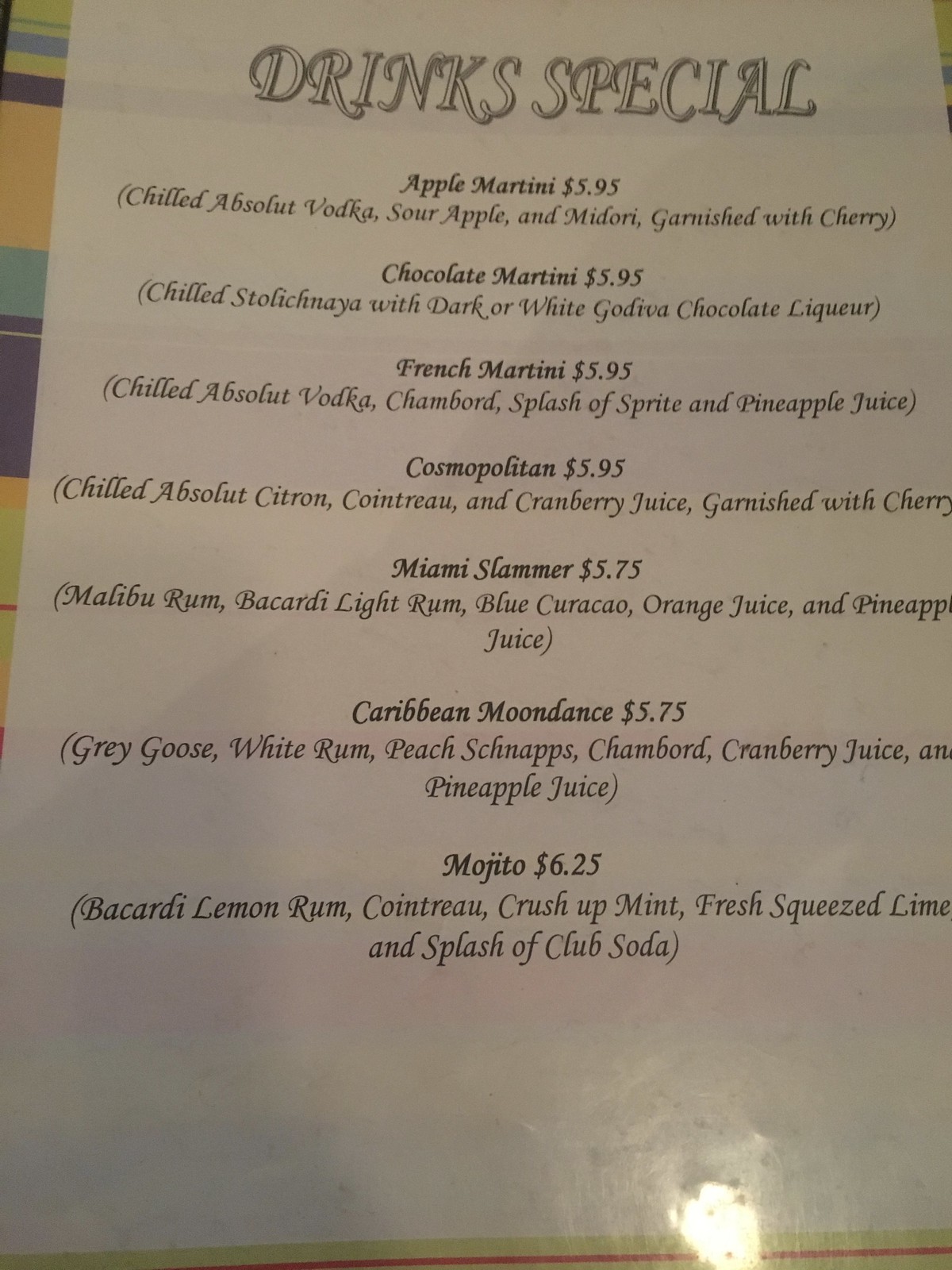**Drinks Special Menu**

This photo captures a zoomed-in view of a drinks special menu, prominently showcased on what appears to be a striped tablecloth. The detailed list of cocktail offerings include the following enticing selections:

1. **Apple Martini** - $5.95
   - Chilled Absolut Vodka
   - Sour Apple
   - Midori
   - Garnish: Cherry

2. **Chocolate Martini** - $5.95
   - Chilled Stolichnaya
   - Dark or White Godiva Chocolate Liqueur

3. **French Martini** - $5.95
   - Chilled Absolut Vodka
   - Chambord
   - Splash of Sprite
   - Pineapple Juice

4. **Cosmopolitan** - $5.95
   - Chilled Absolut Citron
   - Cointreau
   - Cranberry Juice
   - Garnish: Cherry

5. **Miami Slammer** - $5.75
   - Malibu Rum
   - Bacardi Light Rum
   - Blue Curaçao
   - Orange Juice
   - Pineapple Juice

6. **Caribbean Moondance** - $5.75
   - Grey Goose
   - White Rum
   - Peach Schnapps
   - Chambord
   - Cranberry Juice
   - Pineapple Juice

7. **Mojito** - $6.25
   - Bacardi Lemon Rum
   - Cointreau
   - Crushed Mint
   - Fresh Squeezed Lime
   - Splash of Club Soda

The absence of a detailed background brings full attention to the menu, highlighting the appealing and diverse cocktail options available.